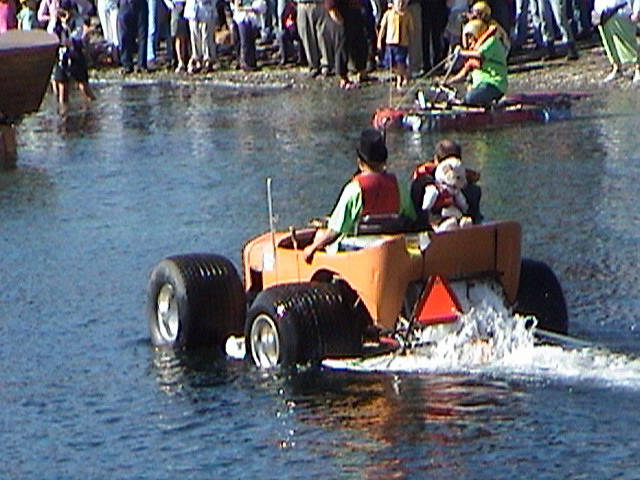This image is a color photograph in landscape orientation, depicting a scene on a lake or another body of water. The main subject in the foreground is a makeshift remote-controlled paddle boat with wide, large tires on either side and a low body painted gold. The vehicle is clearly not a conventional car; it is designed for moving through water, possibly indicating a flood situation or an intentional ride through a lake or river. The operators, who are facing away from the viewer and paddling toward the left side of the image, are seated inside the boat, which leaves a wake of white water behind as it moves to the right. A white stuffed teddy bear is positioned on the back of one of the operators, adding a whimsical touch to the scene. There is also a passenger to the right side of the main operator. In the background, another paddle boat with an operator in a bright green t-shirt is visible, with much of it partially submerged in the water. Distant figures on the shoreline are also seen, their lower halves visible, contributing to the realistic and representational nature of the photograph.